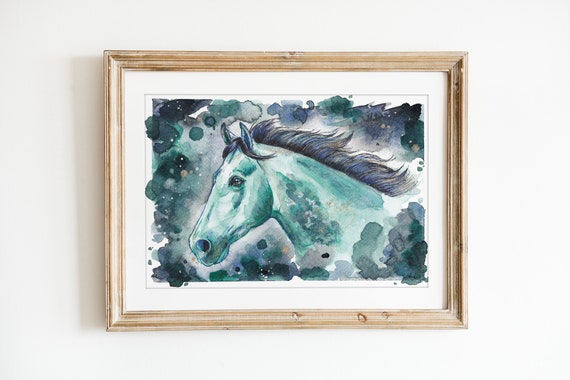The photograph captures a painting hanging on a white wall, centrally positioned. The painting is framed with a light brown wooden frame and features a thick white border, followed by a thinner gray rectangle that frames the main artwork. The focal point of the painting is a side view of a horse's head and neck, facing left, rendered primarily in blue-gray watercolors. The horse's mane flows to the right in shades of bluish and purplish hues. The horse's ears and mane tips are a brownish-black color. The background of the painting is filled with large, cloudy splotches and flecks of abstract colors, including varying shades of green, purplish hues, and some white. These splotches surround the horse, creating a striking contrast against the detailed rendering.